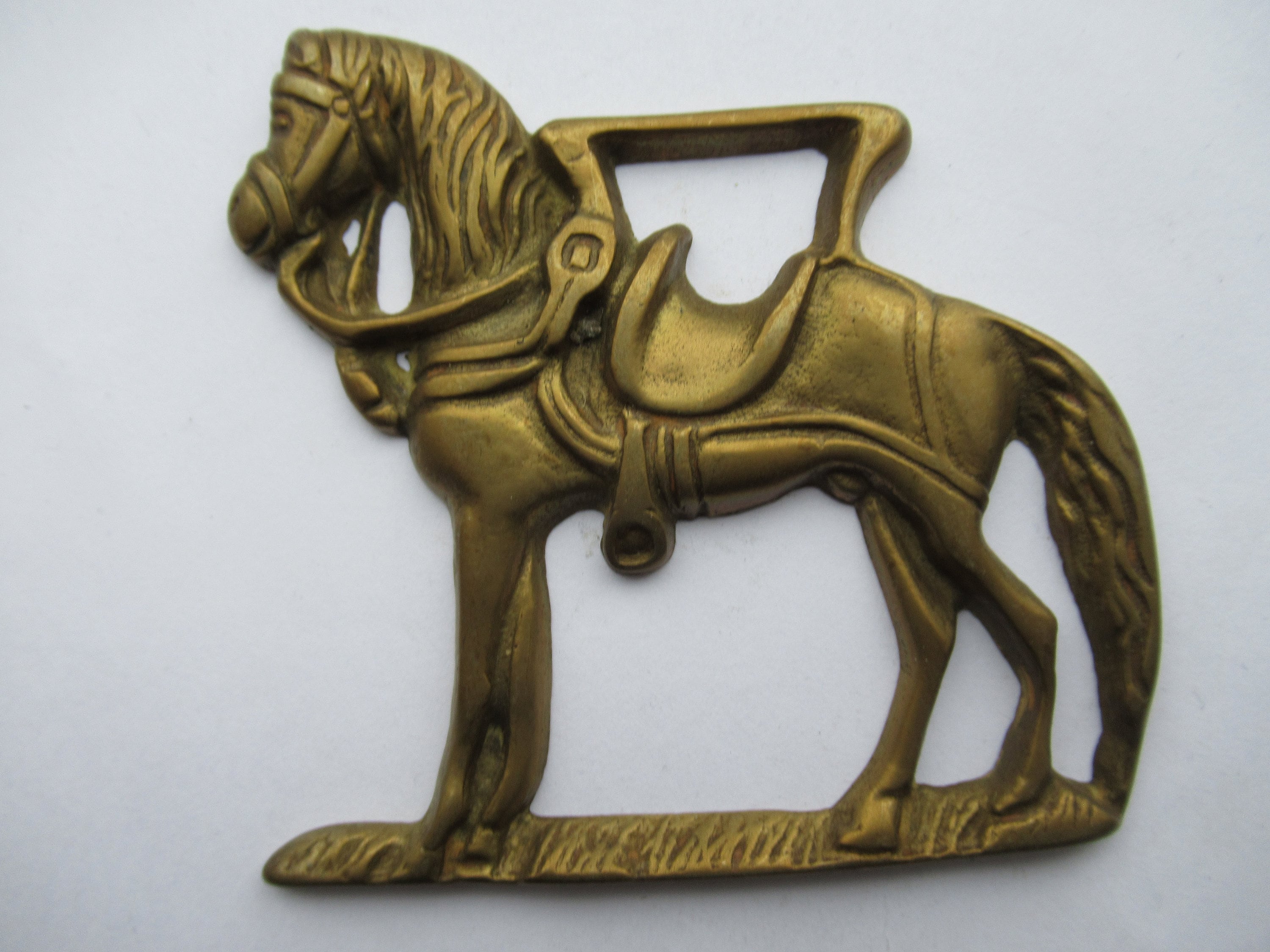The image is a detailed photograph of a small, metallic horse sculpture, seemingly designed as a decorative ornament. The sculpture, which appears to be crafted from bronze or copper or perhaps painted to mimic those materials, is presented in a gold, tarnished hue. The horse stands on a slender, ground-like base and faces left. It is adorned with a saddle and a bridle, with the reins and stirrup clearly visible. The horse’s long mane and tail add to its realistic portrayal. The entire piece, including the handle-like square shape at the top, suggests it is intended for decorative purposes, possibly hung up or placed as a standalone ornament. The sculpture is photographed against a neutral light blue background and does not exceed five inches in height and width, making it a compact yet intricate decoration.